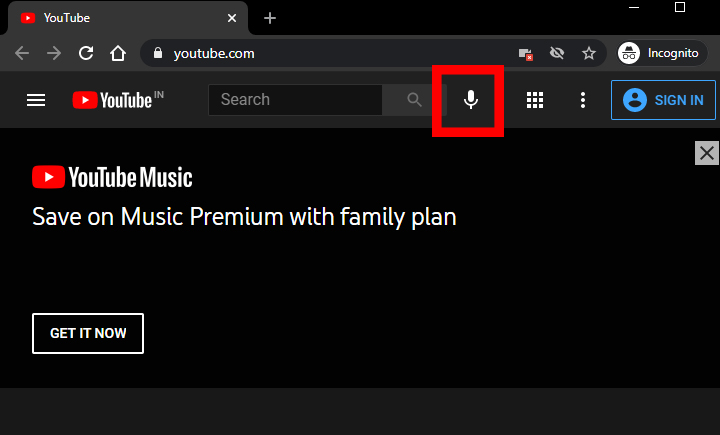This image captures a screenshot of the YouTube website viewed on a computer, featuring the platform's dark theme. The main components of YouTube's interface are in focus, enhanced by a black bar stretching across the top of the screen. On the left side, three horizontal lines signify the menu icon for selecting various options. Adjacent to this menu icon, the iconic red play button logo is visible, followed by the "YouTube" name in white text, accompanied by the letters "I N" slightly above the final "E".

In the middle of the top bar, a search bar is prominently displayed along with a microphone icon to its right. A thick red box is drawn around this microphone, emphasizing the feature for the purpose of the tutorial. Further to the right, a grid icon composed of nine squares offers viewing options for videos, followed by a vertical ellipsis symbolizing the settings menu. There is also a blue link for users to sign in.

Below the primary navigation bar, there is a promotional banner for YouTube Music, highlighting a family plan with the text: "Save on music premium with family plan." At the bottom of the banner, a clickable link stands out with a distinct white outline, black background, and the words "Get it now," inviting users to purchase the YouTube Music premium family plan.